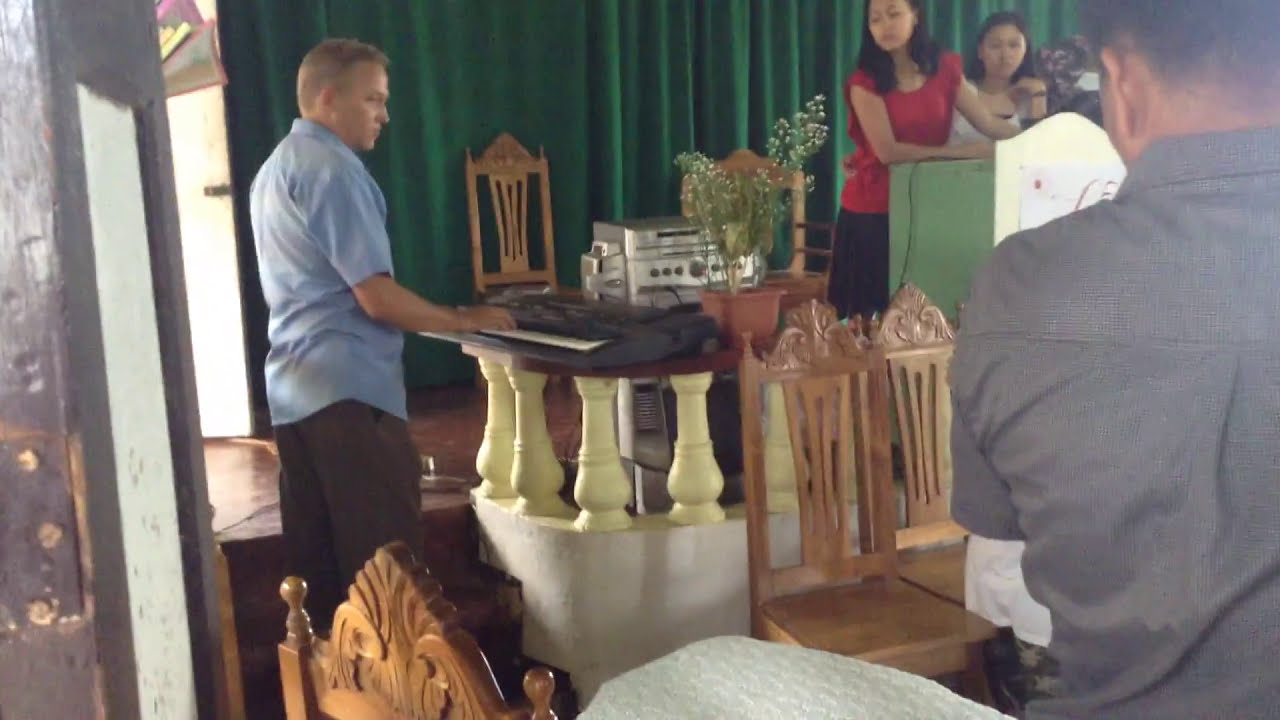In this detailed photograph of an indoor setting, a man dressed in a blue button-down shirt and dark pants is playing an electronic keyboard, which is placed on a set of yellow columns resembling a permanent table structure. The keyboard is situated in front of a stage adorned with dark green curtains. Around the stage area, various pieces of audio equipment and wooden chairs are visible, all appearing as part of a matching set. In front of the stage, standing next to some dried flowers or plants, are three women, one of whom is wearing a red shirt paired with a black skirt and is intently looking at the keyboard player. There is a man with his back towards the camera, dressed in a short-sleeved gray shirt, positioned on the right side of the frame. The space appears cramped, indicating limited room for movement, suggesting that the individuals present are likely focused on listening to the music being played rather than dancing.